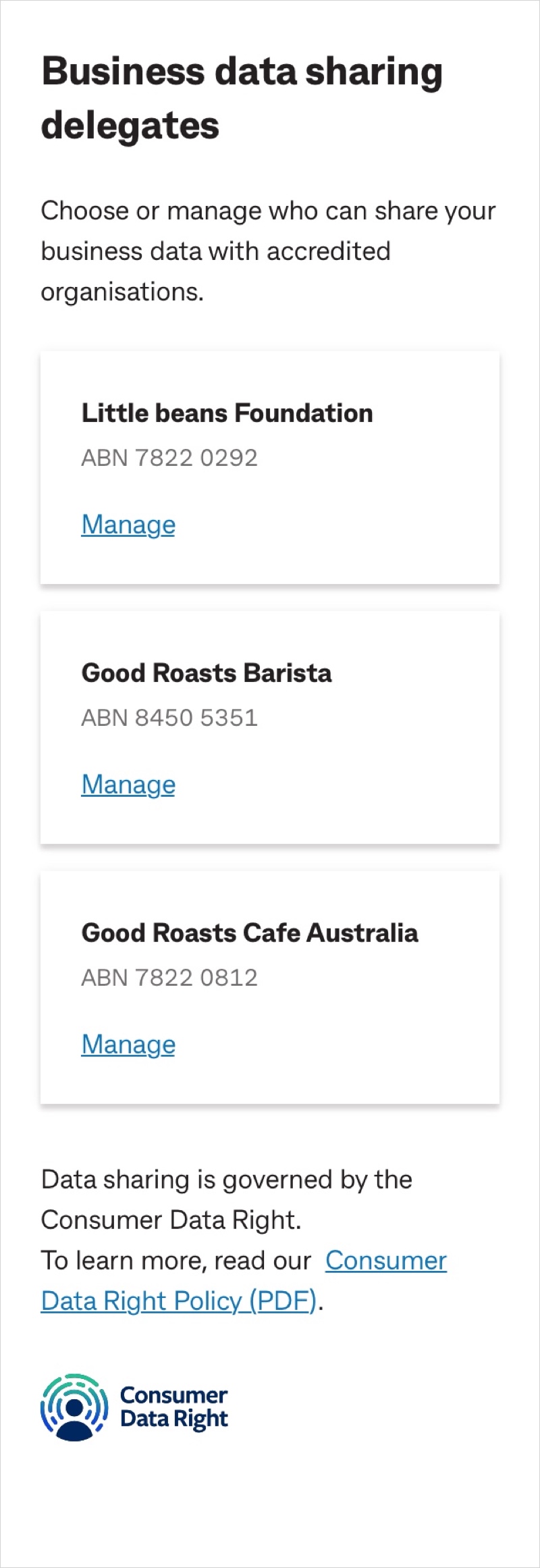This image appears to be a screenshot related to Consumer Data Rights, specifically showcasing a feature for managing business data-sharing delegates. It seems to be part of a website or application interface, although no direct web address or official branding is visible.

At the top, the section mentions its function: "Business Data Sharing Delegates". It allows users to choose or manage which accredited organizations can access their business data. The interface seems structured with multiple tiles representing different organizations, each accompanied by a unique ABN (Australian Business Number) and a "Manage" button.

The first tile features the "Little Beans Foundation" with ABN 7822-0292. Next, there's "Good Roasts Barista" with ABN 8450-5351. The final tile shows "Good Roasts Cafe Australia" with ABN 7822-0812. Each organization has a corresponding "Manage" button for users to control data-sharing permissions.

At the bottom of the image, there's a note emphasizing that data sharing is governed by the Consumer Data Right, directing users to a "Consumer Data Right Policy PDF file" for more information.

The Consumer Data Right logo appears in dark blue and incorporates a simple hand-drawn figure with blue and green elements.

Overall, this interface enables businesses, particularly those potentially related to coffee, to manage their data-sharing settings with specific organizations.